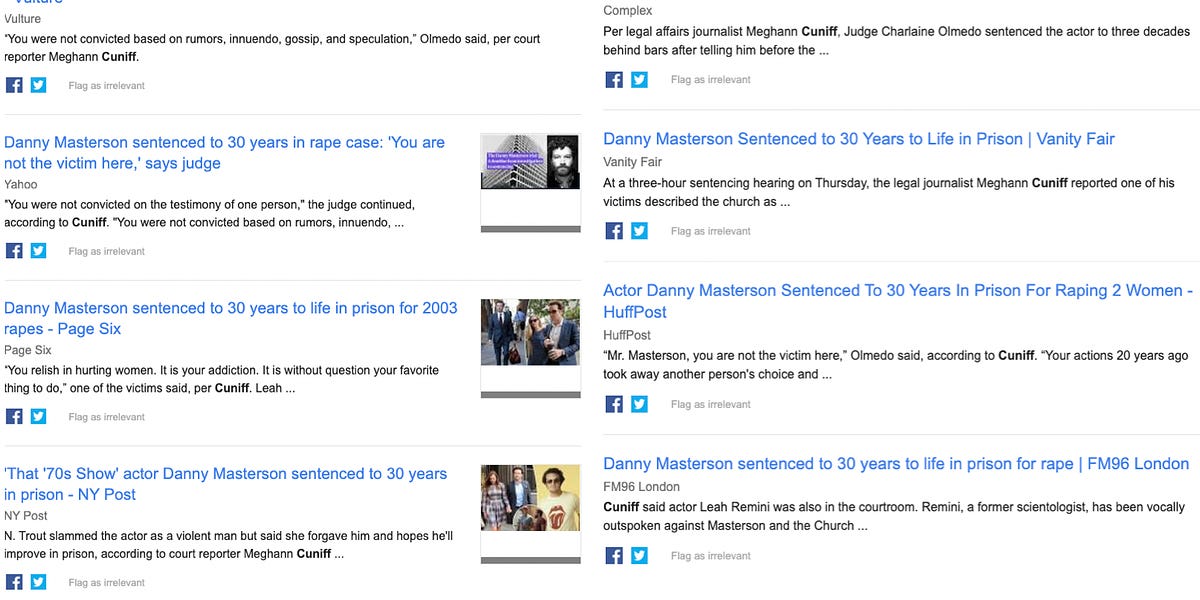**Screenshot of Search Results for Danny Masterson Case**

This screenshot captures eight search results related to Danny Masterson, each detailing the recent sentencing news of the actor. Unfortunately, the titles of the top two results are partly obscured. 

Starting from the left side:
1. **Source: Culture Unspecified** - The title is not visible, but the snippet quotes Almeida, as reported by court reporter Megan Cuniff, stating, "You were not convicted based on rumors, innuendo, gossip, and speculation." Each result includes symbols for sharing on Facebook and Twitter, and a notice reading "flag as irrelevant."
   
2. **Source: Yahoo** - The headline states, "Danny Masterson sentenced to 30 years in rape case. 'You are not the victim here,' says judge." It continues with another quote, "You were not convicted on the testimony of one person," as emphasized by Cuniff. This entry features a small photo on the right depicting a building with purple text alongside an image of Danny Masterson.

3. **Source: Page Six** - The result reads, "Danny Masterson sentenced to 30 years to life in prison for 2003 rapes." It includes dramatic victim statements, "You relish in hurting women. It is your addiction. It is without question your favorite thing to do," as noted by Cuniff. This entry includes two photos, presumably of Masterson.

4. **Source: New York Post** - Headlined, "That '70s Show actor Danny Masterson sentenced to 30 years in prison," it reports that N. Trout called Masterson a violent man while adding that she forgave him and hopes he'll improve in prison, once more citing Megan Cuniff.

On the right side:
1. **Source: Complex** - This entry titles, "Pro-legal affairs journalist Megan Cuniff: Judge Charlene O'Neill sentenced the actor to three decades behind bars," detailing the courtroom proceedings.

2. **Source: Vanity Fair** - It mentions, "Danny Masterson sentenced to 30 years to life in prison," focusing on a three-hour sentencing hearing with reports from legal journalist Megan Cuniff, including a victim's description related to the church.

3. **Source: HuffPost** - The headline states, "Actor Danny Masterson sentenced to 30 years in prison for raping two women," reiterating, "Mr. Masterson, you are not the victim here," with further commentary by Cuniff on the impacts of his actions.

4. **Source: FM96 London** - The result echoes, "Danny Masterson sentenced to 30 years to life in prison for raping," reporting that actor Leah Remini, also present in the courtroom, has been vocally critical of Masterson and the Church of Scientology.

All results are presented in black text with their titles highlighted in blue, providing various perspectives and details on the high-profile sentencing of Danny Masterson.